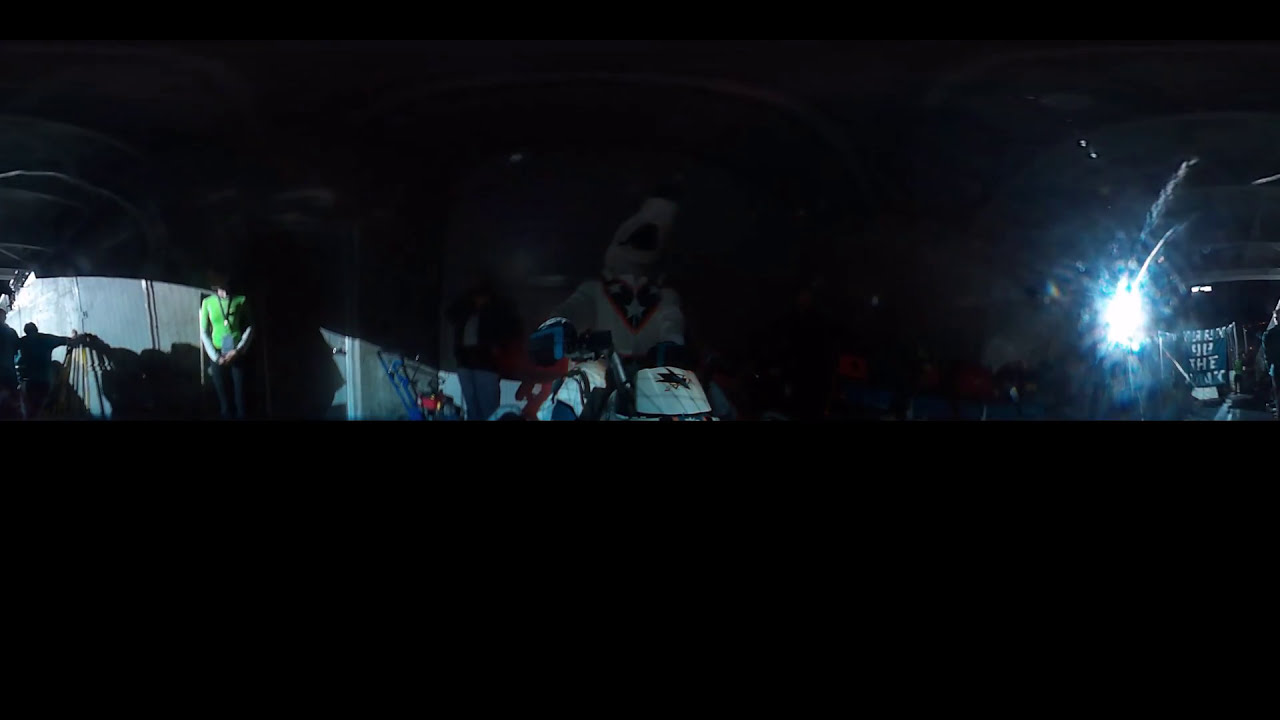The image is predominantly a dark, outdoor urban scene captured in a photographic style, seemingly through a car window, indicated by a light glare on the right side. The center of the image is illuminated as though by a splash of light, highlighting different elements against the backdrop of near-total darkness. 

To the left, there is a man, head out of frame, wearing a green shirt and dark blue jeans, with a lanyard around his neck. He stands in front of a grayish-blue metallic door with a yellow handle, adjacent to a concrete wall adorned with graffiti of a clown. Just left of this man, a second person in a wheelchair is visible, descending a ramp. 

Graffiti marks the wall right of the door, beneath which a toy truck is positioned. Further to the right, a red and white scooter is parked on the street. In addition, a dimly visible billboard towards the right of the frame contains an ambiguous message with words like "Virgin" and "day" faintly discernible. An overall dark horizontal bar blankets the bottom 40% of the image, accentuating the stark contrast and directing focus towards the selectively lit subjects and surroundings.